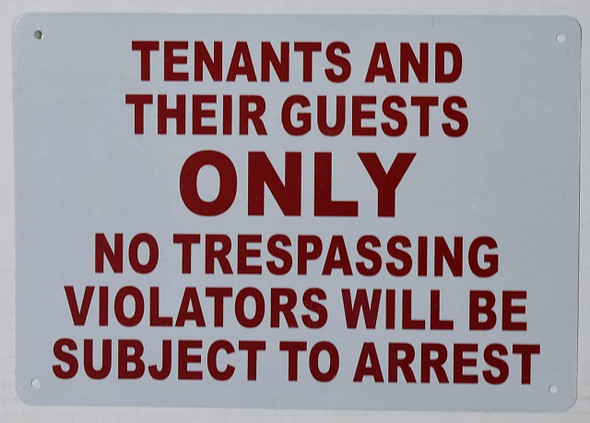This is a color photograph of a metal or tin sign set against a light gray, solid background. The sign is a plain gray or very light blue color with four holes, one in each corner, presumably for mounting. The bold, all-capital text on the sign is maroon or red, with the word "ONLY" significantly larger than the rest. The message on the sign reads in descending order: "TENANTS AND" on the first line, "THEIR GUESTS" on the second line, "ONLY" on the third, "NO TRESPASSING" on the fourth, "VIOLATORS WILL BE" on the fifth, and "SUBJECT TO ARREST" on the sixth line. The sign appears to be slightly wider than it is tall, suggesting it could be mounted on a building, possibly at a residential complex, to restrict access to tenants and their guests only.